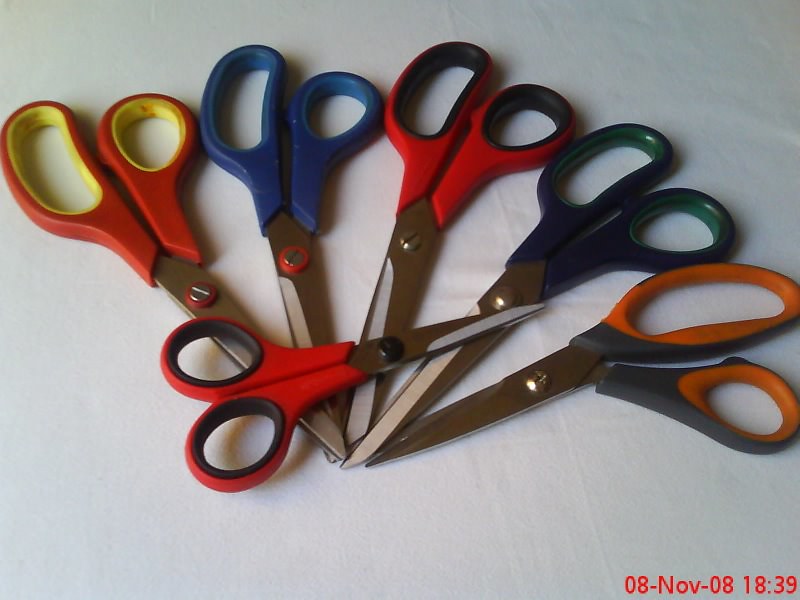This is a detailed landscape photograph taken on 8th November 2008, at 18:39. The image features six pairs of scissors, arranged meticulously on a white fabric background with visible creases. Five of the scissors fan out from a central point, creating an arc with their handles. The scissors, from left to right, are identified by their distinct handle colors: red with a yellow interior, blue, red with a black interior, blue with a green interior, and gray with an orange interior. Each handle points outward towards the edges of the photograph, and their tips converge at the center, slightly overlapping. In contrast, a smaller pair of scissors, with red handles and a black interior, lays horizontally atop the arc, intersecting the others at a slight 30-degree angle from the mid-right to the left. This vibrant and orderly composition of scissors on the textured white backdrop presents a striking and colorful visual.